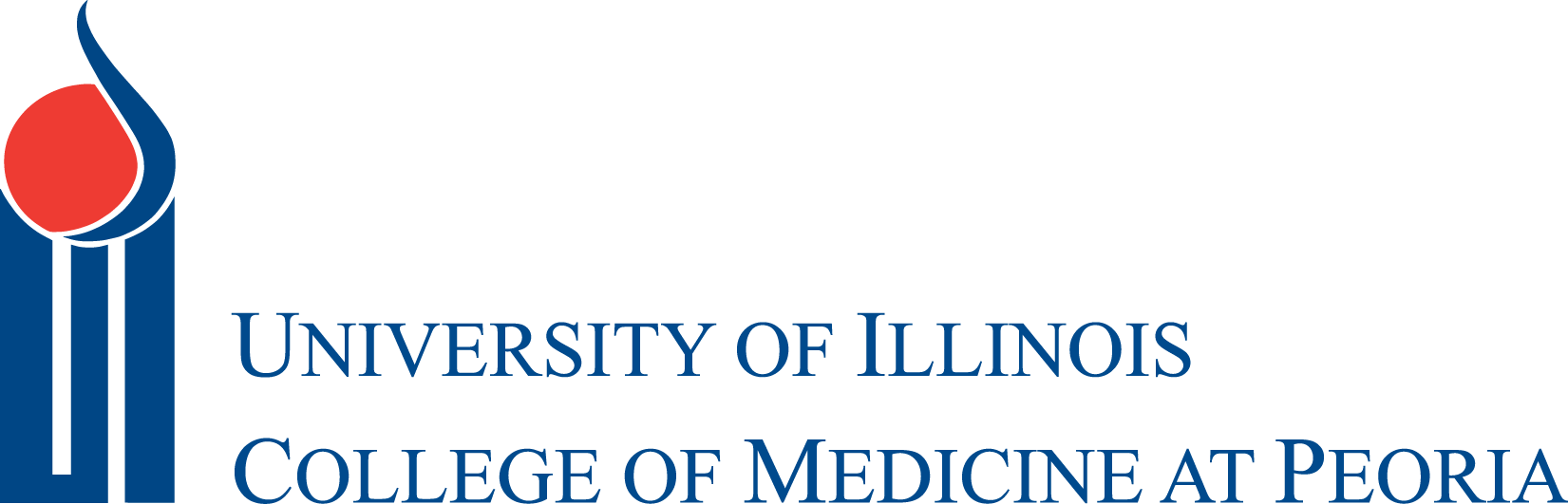This digital image features the logo of the University of Illinois College of Medicine at Peoria. The logo is set against a clean, white background. The main text, written in a dark blue serif font, is composed of two lines: "University of Illinois" on the first line and "College of Medicine at Peoria" on the second, both left-justified. To the left of the text, there is a visual emblem consisting of the initials "U" and "I" in a tall, narrow, and very bold font, resembling skyscrapers. Above these initials, there is a bright red circle framed by a blue curve that extends from the bottom right, up and around the right side of the circle, and then continues upward. This red circle and blue curve are outlined in a thin white line, adding definition to the shapes. The text in the logo is entirely in capital letters, with the first letter of each word slightly larger than the remaining letters in that word, providing a sense of hierarchy and emphasis.